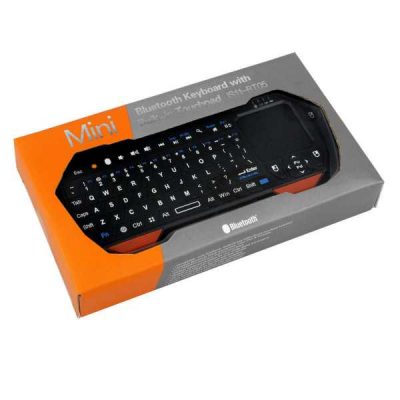The image showcases a compact box divided into two color segments: an orange section on the left and a gray section on the right. Encased within the box is a mini Bluetooth keyboard. The orange part of the box prominently displays the word "mini," while the gray part features the phrase "Bluetooth keyboard," though some text is slightly blurred. The model number "IS11-R105" is also visible. At the bottom, the word "Bluetooth" accompanied by its iconic symbol stands out in bright white.

The box's side is detailed with about seven fine lines of text, likely outlining the device's specifications. The keyboard itself adheres to the QWERTY layout, featuring the keys Q to P in the top row, A to L in the middle row, and Z to M in the bottom row. Special characters such as less than (<), greater than (>), comma (,), period (.), question mark (?), and slash (/) are also present on the right side of the keyboard. The top row includes number keys from 1 to 0 and additional keys for plus (+), minus (-), slash (/), parentheses (()), and other symbols. Function buttons are notably highlighted with a mix of orange and white icons.

Interestingly, there is a small screen on the right-hand side of the keyboard, which appears to function as a drawing surface. This versatile mini keyboard seems ideal for use with a variety of remote devices.